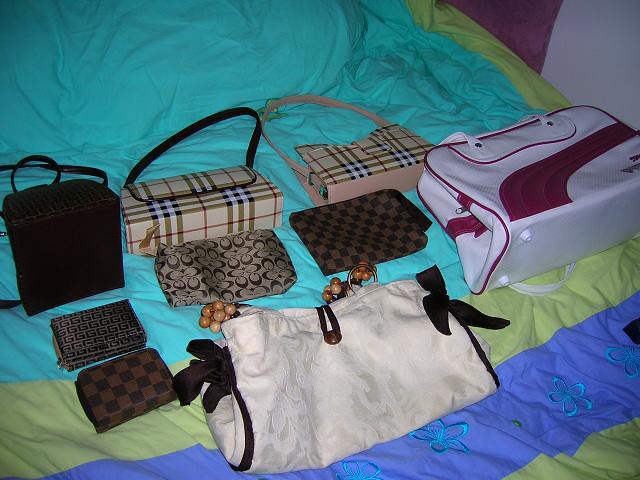This rectangular photograph showcases a meticulously arranged collection of luxury handbags and wallets spread out on a vividly colored comforter with blue, green, and purple stripes, accented by appliques of flowers. Dominating the display are two Burberry-style plaid handbags positioned prominently at the top. In the center, a black Coach wallet is flanked by an assortment of other small wallets, totaling four. Also included in the collection are two medium-sized makeup bags. On the right side, there's a white handbag with brown trim, a distinctive Puma bowling bag, and a hint of brown beaded jewelry adding an extra touch of elegance. Meanwhile, the left side features another large black handbag and additional unbranded bags below. The vibrant setting contrasts beautifully with the mixed patterns and colors of beige, lavender, pink, brown, and black bags, all artfully arranged on a teal blue bedsheet.